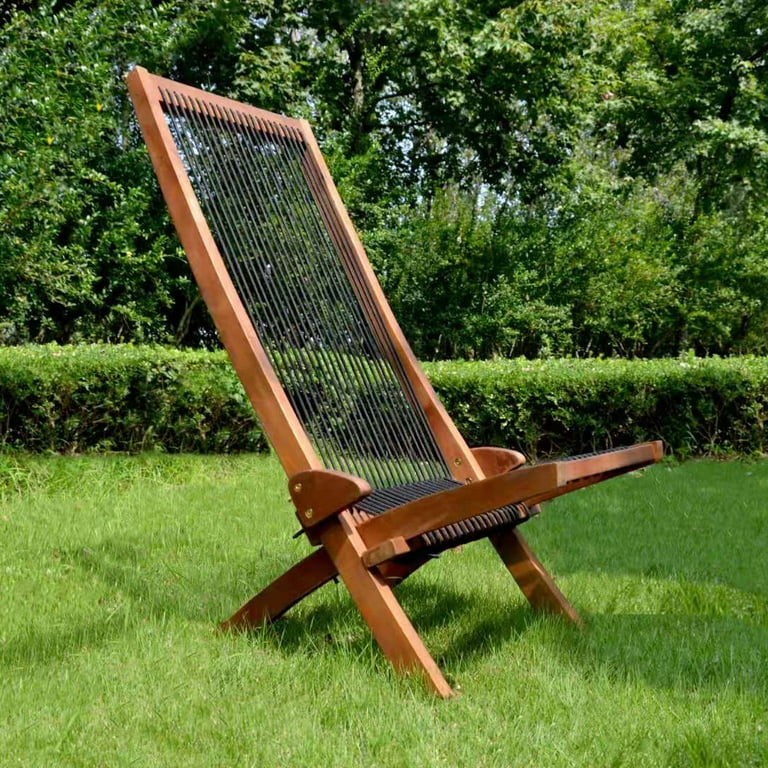In this daytime outdoor image, the backdrop features a bright, open sky partially obscured by a canopy of tall, deciduous trees fully leafed out in vivid green. Beneath these trees, a layer of various shrubs and bushes adds depth to the scene. The lower level of the garden reveals meticulously trimmed, low-growing bushes stretching along the forefront, complemented by a lush, healthy green lawn.

Amongst this verdant setting, there stands a distinctive wooden weaving machine. At first glance, it might be mistaken for an unconventional chair due to its intricate design. The frame is brown, with tall back support and legs that form an X-shape at the bottom. Instead of a traditional seat and backrest, the machine is strung with taut black lines, resembling either shoelaces or bungee cords. These details highlight the unique craftsmanship and intriguing aesthetic of the weaving machine, set against the natural splendor of the landscaped garden.